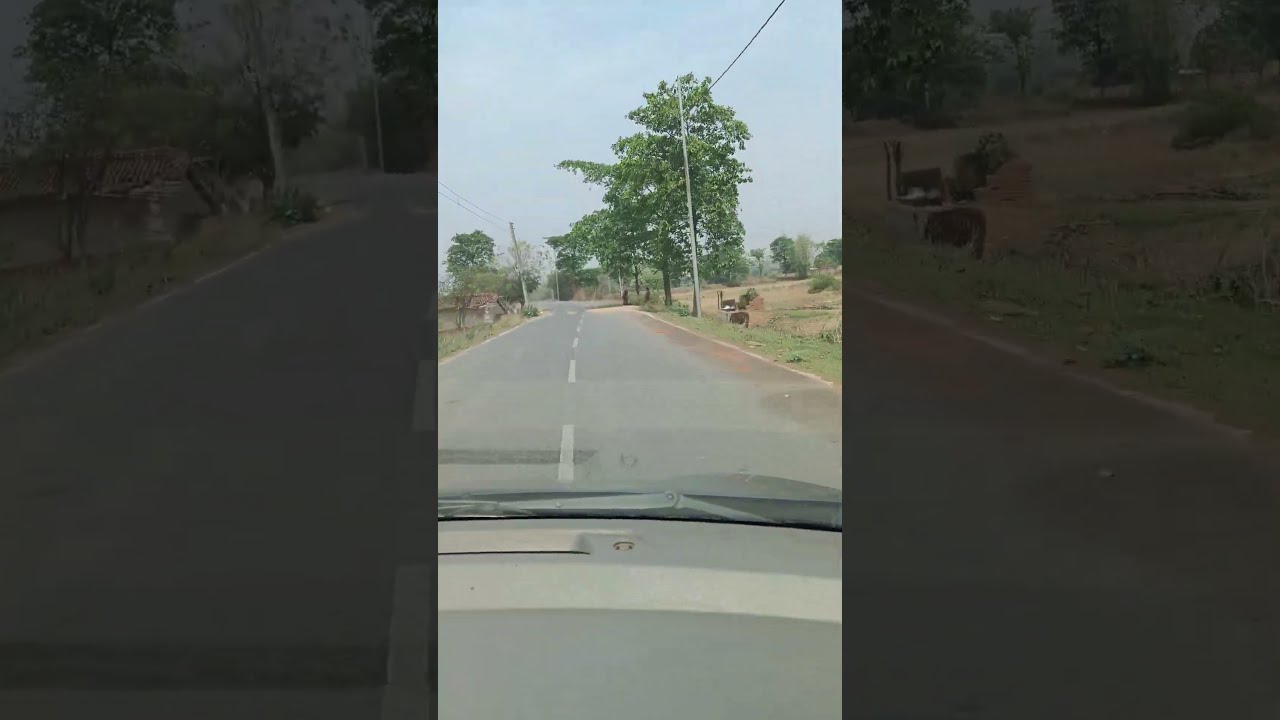The image is a detailed color photograph taken from the inside of a car, looking out through the windshield at a light gray road with a dotted white line running down its center. The sky is a clear blue with a few clouds. Sparse trees and green fields with cattle flank either side of the road, which appears to curve slightly to the left in the distance. Power poles line the road, adding to the serene, rural landscape. 

This central portrait image is framed by two darker, out-of-focus, and enlarged vertical segments on either side, which are essentially blown-up and darkened details of the main image. These side panels create an elongated landscape format, contrasting the sharp details of the central road scene with their black, opaque backgrounds.